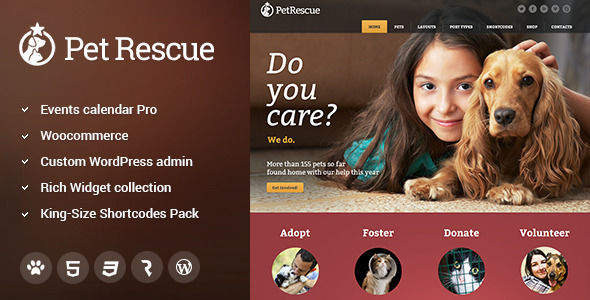This is a detailed descriptive caption for an image of a pet rescue website:

---

This image is a snapshot of a pet rescue website, featuring a visually organized layout with distinct sections and vibrant detail. The left side of the page has a vertical rectangular box with a brown background, prominently displaying the words "Pet Rescue" in white lettering. Below the heading, the section contains five check marks followed by text descriptions: "Events Calendar Pro," "WooCommerce," "Custom WordPress Admin," "Rich Widget Collection," and "King Size Shortcodes Pack."

Directly beneath these descriptions, there are five light brown circles with white text symbols. The first circle displays a paw print, the second has the number five, the third contains the number three, the fourth features a partially shown question mark, and the last one shows the letter W.

On the right side of the website, there is a horizontal rectangular section featuring an image of a young girl with long brown hair lying on the floor beside a tan cocker spaniel. Accompanying this picture is the text, "Do you care? We do. More than 155 pets so far found homes with our help this year."

Below this section is another rectangular box, this time red in color, containing the calls to action: "Adopt," "Foster," "Donate," and "Volunteer." In this area, there are also four circles, each showcasing images of cats, dogs, or people engaged in rescue activities.